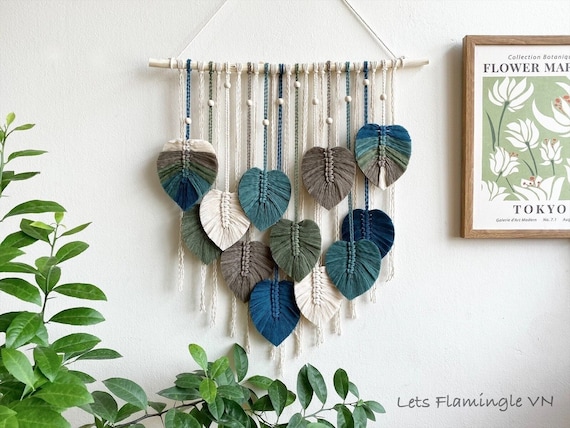The image displays a craft flower wall hanging on an off-white wall. The top portion, where the hanging presumably attaches with a pin or nail, is out of view. Two strings descend from a horizontal, bone-colored rod, supporting an array of hand-made flowers that hang on alternating white and green ropes. These flowers, possibly made from fabric or another craft material, come in shades of light blue, dark blue, white, and brown, contributing to an overall earthy and soothing palette.

To the right side of the hanging, partially cropped out of the frame, is a wooden picture frame containing an illustration of white flowers on a green background with hints of pink. Above the illustration, partially visible text reads "collection, botany, flower ma..." with "Tokyo" underneath it in black font. Below this frame, another wooden sign reads "Let's Flamingo the End," written in a script-like font. To the left of the craft hanging, there is a large potted plant with dense green leaves resembling bay leaves.